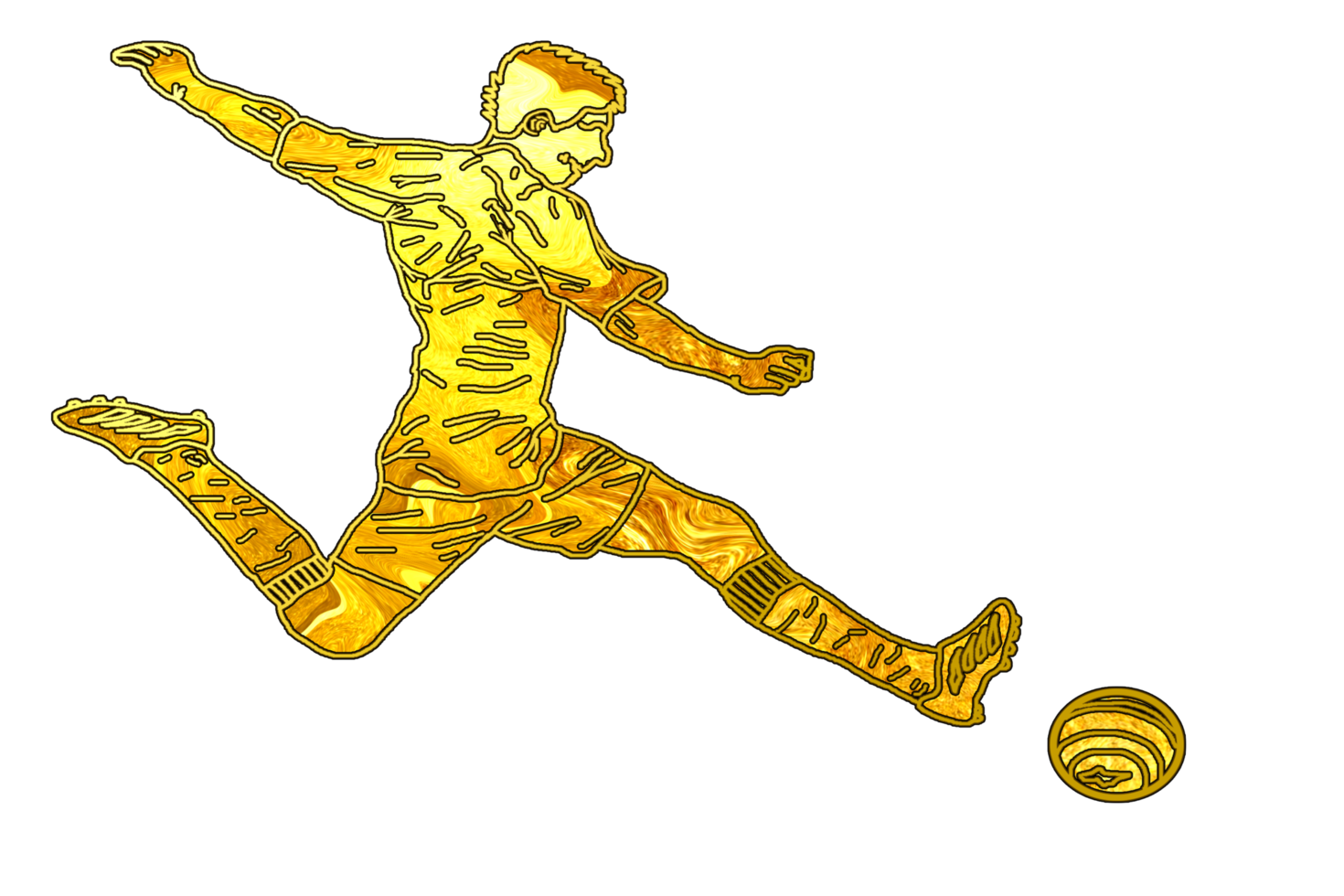The image depicts a stylized, simplistic line drawing of a soccer player in motion, captured at the moment just before kicking a ball. The entire image, including the soccer player and the ball, is rendered in varying hues of yellow, ranging from bright yellow to a golden brown. The background is entirely white, giving the impression of a cutout or a sticker. The soccer player is shown in profile, facing toward the right side of the image, with his arms outstretched and one leg extended as if about to strike the ball positioned in the bottom right corner. The depiction is minimalistic, with simple lines and a flat, almost painted appearance. Details such as the soccer player's cleats, socks, shorts, and hair are all illustrated with subtle variations in the golden-yellow palette, and the ball features stripes that swirl to give it definition. The overall design exudes a warm, golden, fiery aesthetic, making it look like a potential logo or emblem due to its vibrant and striking color scheme.